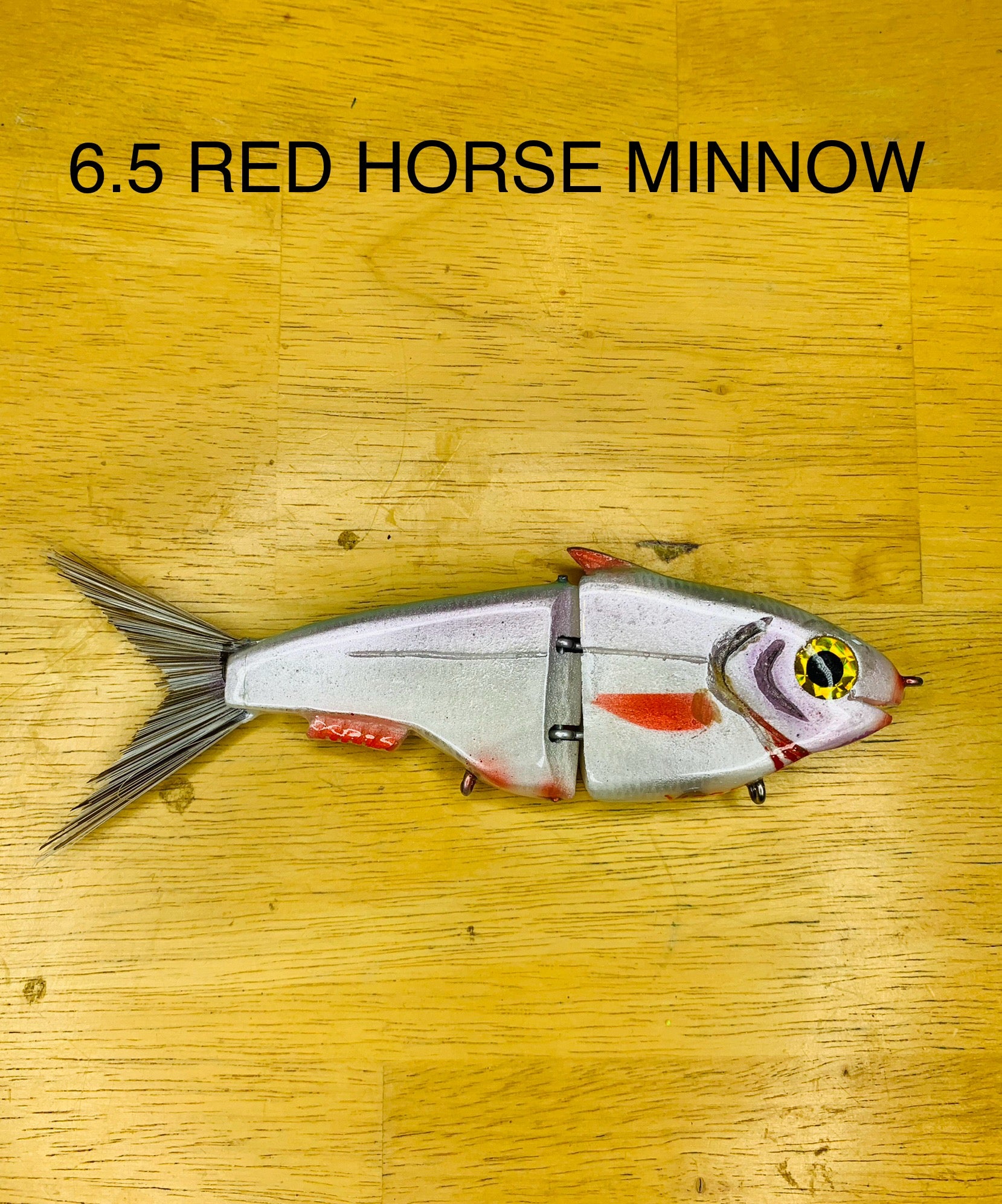This full-color, digitally-enhanced photograph, taken indoors, features a close-up of an old, metallic fishing lure resting on a light, honey-colored wooden surface that might be a cutting board or a table. The vertically rectangular image has black, all-capital text at the top reading "6.5 Red Horse Minnow." The centrally positioned, detailed fishing lure mimics a fish, oriented from left to right. The lure, predominantly gray and metallic, is highlighted with red fins on its side, top, and beneath its tail fin. It has a rear fin that's a darker shade of gray. The lure also features a shiny yellow eye with a black pupil and several small black balls, likely for noise, positioned on its body, including one just above the mouth. Three loops are visible: one at the snout, one under the gills, and one towards the rear body.